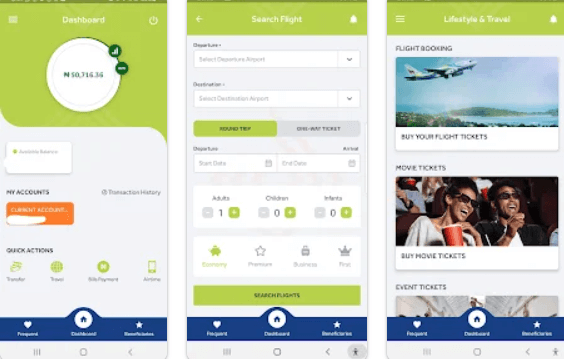Here is a cleaned-up and detailed caption:

---

The image displays three vertically aligned screens with various user interface elements:

**Left Screen:**
- **Top Bar:** A dark green bar at the top.
- **Main Area:** 
    - Contains a speech bubble-like shape with text in yellow and several symbols at the top.
    - A white circle with a thin green outline, featuring green circles along its perimeter.
    - Below, there's a gray shape resembling an upside-down speech bubble with a white rectangle inside.
    - Text beneath it reads "My Accounts" and features an orange rectangle with text and a feather-like white symbol.
    - Additional text in blue and green, which is unclear.
    - Further down, a dark blue rectangle with a middle bulge showcasing a white heart, a white circle containing a blue element, and a white star, with text below these icons.

**Middle Screen:**
- **Top Bar:** Dark green with a thin line.
- **Main Area:** 
    - A lighter green rectangle with a left-pointing arrow and "Search Flight" written next to a bell icon on the left.
    - A large gray rectangle containing indecipherable text.
    - Two white rectangles with downward-pointing arrows on the right, featuring small, unreadable text.
    - A green rectangle with unreadable text adjacent to a slightly darker gray rectangle.
    - Sequence of white rectangles with words and symbols in them, including green elements, which are not legible.
    - Another white rectangle where the first symbol is green, the rest gray, and a green rectangle with unreadable text.
    - A blue rectangle with a middle bulge containing a white heart, a white circle with a blue element, and a white star.

**Right Screen:**
- **Top Bar:** A thin dark green line.
- **Main Area:** 
    - Lighter green section with yellow text and symbols.
    - The text reads "Flight Booking," followed by an airplane icon and text underneath (unreadable).
    - Next section labeled "Movie Tickets" with an icon of people watching a movie and text reading "Buy Movie Tickets."
    - "Event Tickets" showing a partially visible image, obscured by a blue rectangle with a bulge in the middle containing a white heart, a white circle with a blue element, and a white star.
    
---